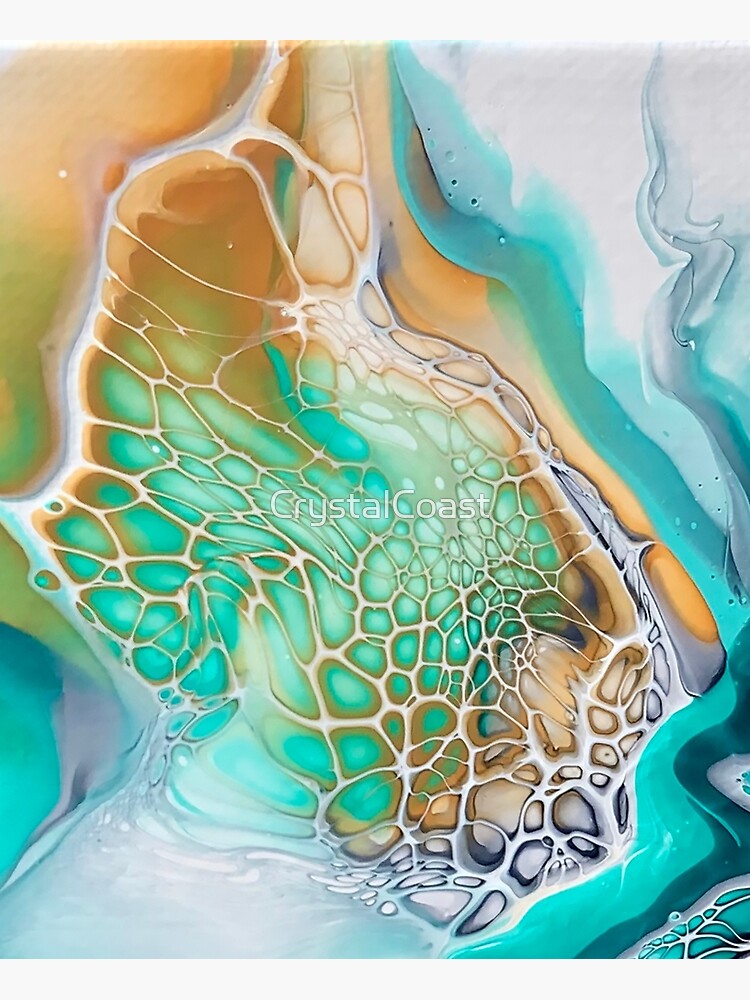This image is a detailed, abstract drawing that could be mistaken for a microscopic view of a cell or tissue. The background is aqua blue, interspersed with various colors and shapes. The top left corner features an orange and rust hue with a large curving cell wall, while the bottom right showcases blue-green cells encased in yellow-beige walls, against a white background with pink, pebble-like elements. Lavender and aqua tones dominate the right side, with darker shades toward the bottom right and lighter hues at the upper right and bottom left, creating a marbled effect. In the center, faint white text reads "Crystal Coast," adding to the artwork's fluid and airy ambience. The varying colors and abstract forms evoke the feeling of water, reminiscent of pour art techniques.